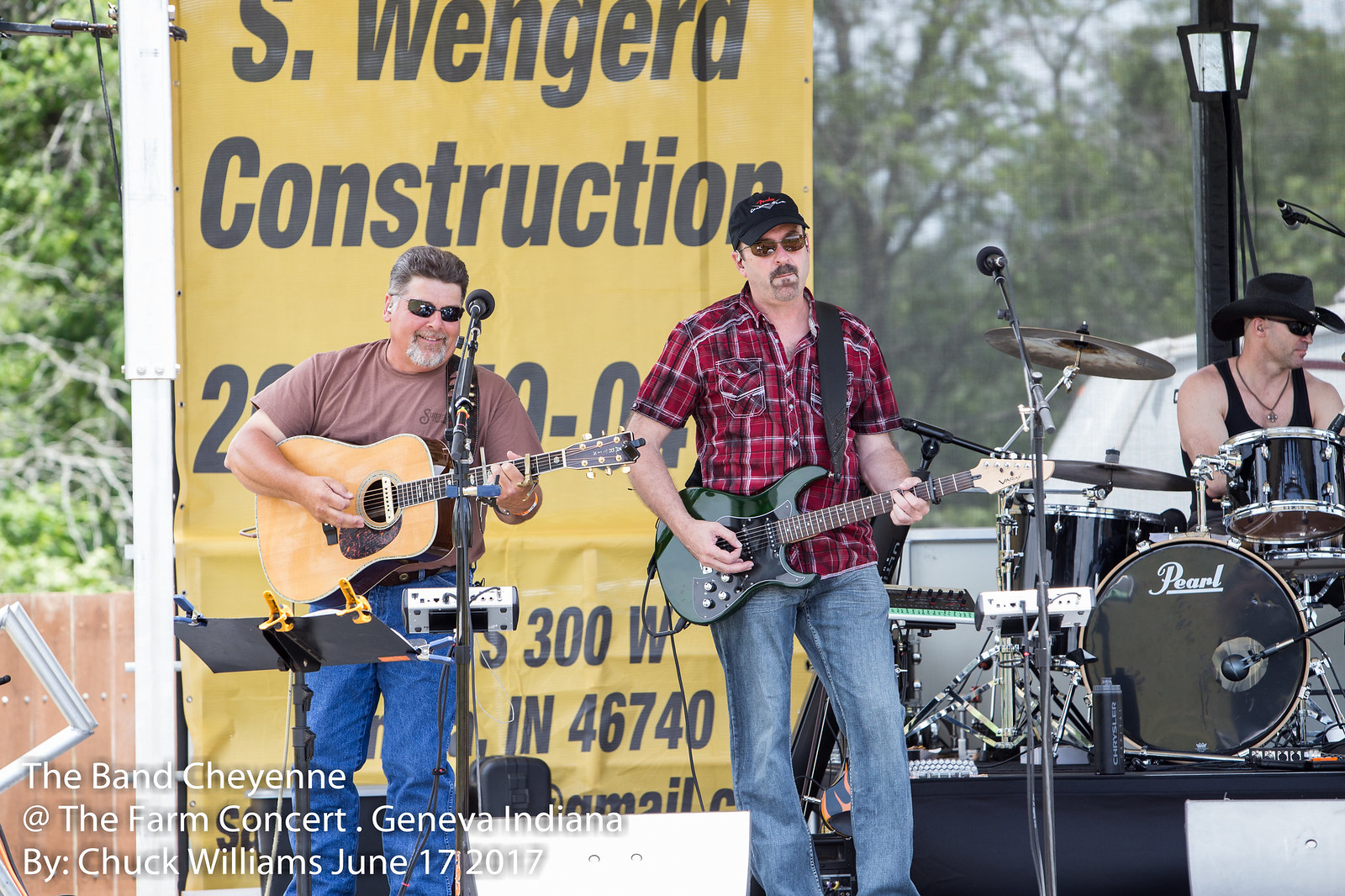In this vibrant outdoor photograph, a band is captured performing on a stage during a daytime festival, surrounded by trees and a fenced area. The background features a light post, part of a vehicle, and a noticeable yellow sponsor banner reading "S. Wengera Construction." The stage setup includes microphones and a music stand. On the left, a man with a white goatee, dark slicked-back hair, and sunglasses strums an acoustic guitar made of beige-colored wood. He is dressed in a brown t-shirt and blue jeans. Centrally positioned, another man in his 30s, clad in a red and black plaid shirt, blue jeans, a black baseball cap, and sunglasses, passionately plays a sleek black electric guitar. He sports a mustache and a goatee. On the right side, a drummer in a black tank top and black cowboy hat, also wearing sunglasses, is energetically performing on a drum set elevated on a podium. The left bottom corner of the image has white text reading, "The band Cheyenne at the farm concert, Geneva, Indiana, 2017."